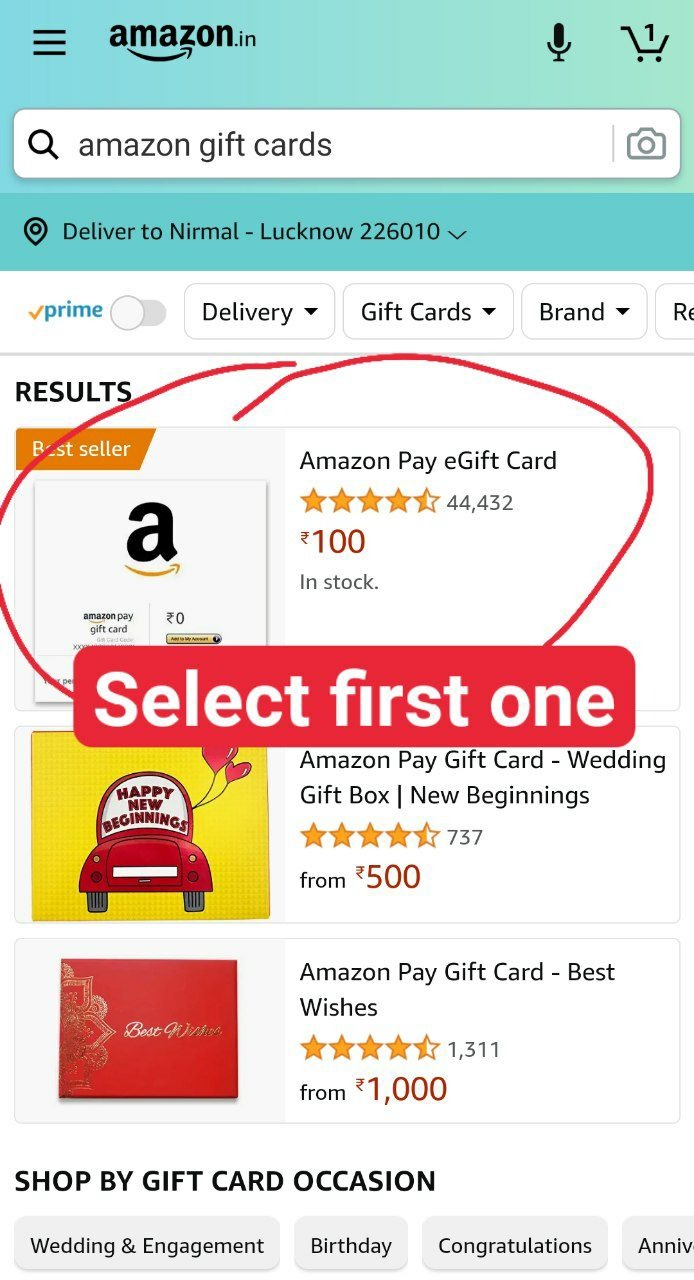This caption contains a detailed description of a partial mobile screenshot from Amazon India's webpage, specifically showcasing the search results for Amazon gift cards.

---

**Partial Mobile Screenshot of Amazon India’s Gift Cards Search Results**

The screenshot captures a section of Amazon India's mobile webpage. At the very top is the header, featuring a search box with the keywords "Amazon gift cards." Directly underneath, there are navigation tags labeled: "Delivery," "Gift Cards," "Brands," and a toggle button for Amazon Prime.

This image displays the first three results on the search page. 

1. **First Result**:
    - **Type**: Amazon Pay E-Gift Card
    - **Rating**: 4.5 out of 5 stars
    - **Reviews**: 44,432 reviews
    - **Price**: Approximately $100
    - **Availability**: In stock
    - **Label**: Bestseller (highlighted in orange)
    - **Annotation**: Circled in red with a red speech bubble saying "select first one"

2. **Second Result**:
    - **Type**: Amazon Pay Gift Card, Wedding Gift Box - New Beginnings
    - **Rating**: 4.5 out of 5 stars
    - **Reviews**: 737 reviews
    - **Price**: Starts from $500
    - **Image Description**: A red car with "Happy New Beginnings" written on the windshield, accompanied by two heart-shaped balloons on the right side.

3. **Third Result**:
    - **Type**: Amazon Pay Gift Card, Best Wishes
    - **Rating**: 4.5 out of 5 stars
    - **Reviews**: 1,311 reviews
    - **Price**: Starts from $1,000
    - **Image Description**: A red box with "Best Wishes" emblazoned in gold and a floral design in gold adorning the left edge of the box.

Below these search results is a section titled "Shop by Gift Card Occasion," featuring three visible tags: "Wedding and Engagement," "Birthday," and "Congratulations."

In the upper right corner of the header is a shopping cart icon with a numeral "1" inside it, indicating one item in the cart. To the left of the shopping cart is a microphone icon.